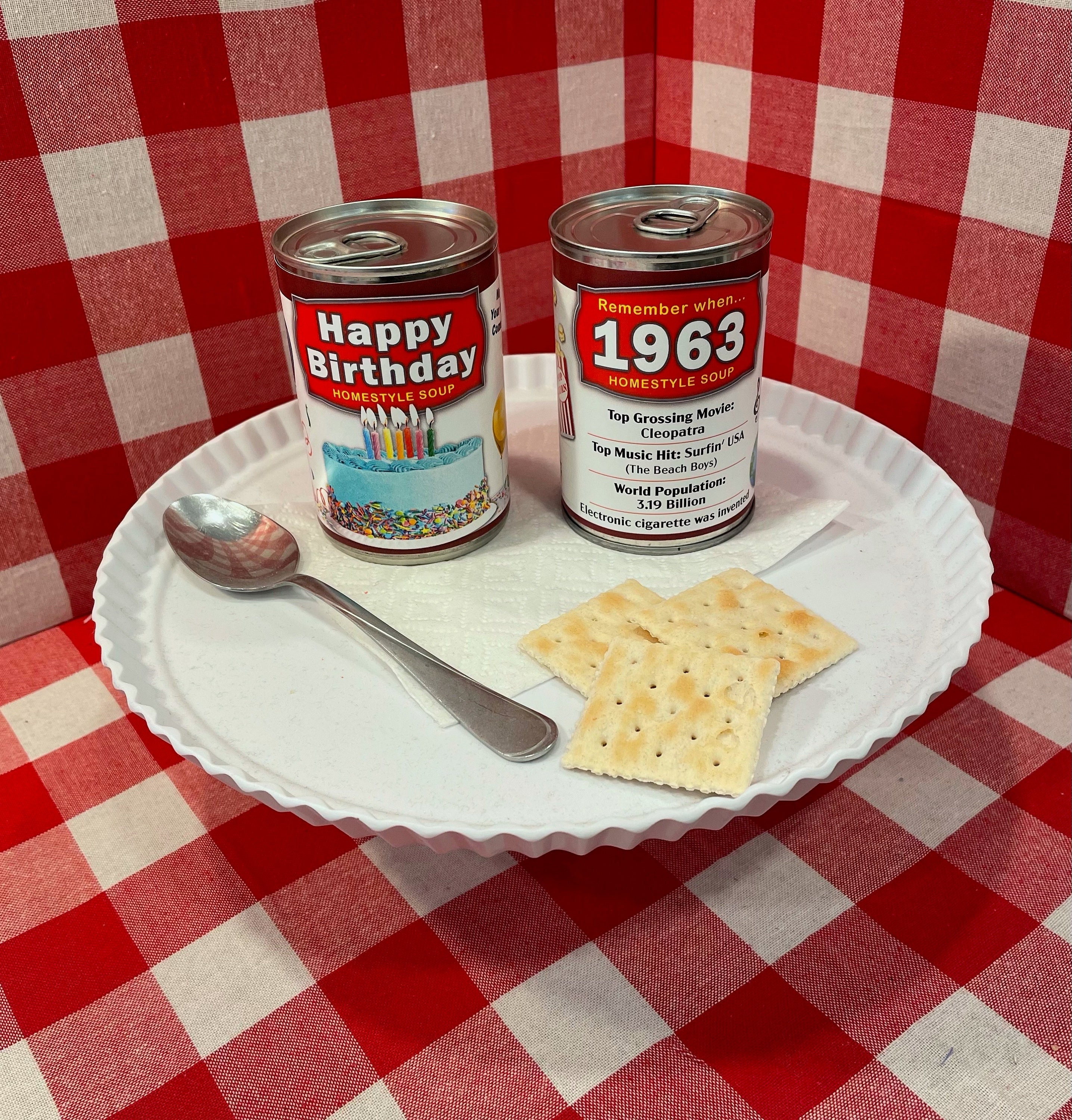The image depicts a detailed and nostalgic tabletop setting. A large, white fluted plate sits at the center, set against a red and white gingham fabric backdrop, which covers both the wall and tabletop, creating a cohesive and festive atmosphere. On the plate, a white napkin serves as the base for an arrangement of items. 

Two cans of soup are prominently placed on the napkin. The first can is decorated with a celebratory "Happy Birthday" message in white letters against a red background, featuring a blue birthday cake with candles illustration. The second can is a nostalgic "Remember When 1963" Homestyle Soup, with a large "1963" in white letters on a red label. The can also features trivia from 1963, highlighting the top grossing movie "Cleopatra," top music hits like "Surfin' USA" by The Beach Boys, and notable facts such as the global population of 3.19 billion and the invention of the electric cigarette.

To the left of the cans, a silver spoon is placed, and in front of it, three saltine crackers are neatly layered. This all sits on the large white fluted plate, which enhances the vintage and charming presentation. The overall composition is thoughtfully arranged, evoking a sense of nostalgia and celebration.